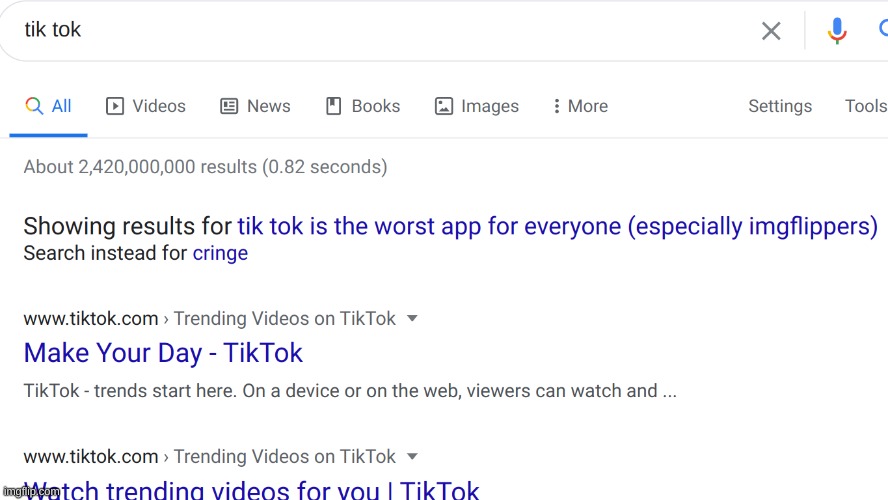The image depicts a Google search results page. At the top, the search bar is visible in a long rectangular shape. On the far left of the search bar, the words "Tick Tock" are written in black text. On the far right, there is a gray 'X' symbol, a microphone icon that is blue on the top half and red, yellow, and green on the bottom half, and a magnifying glass icon.

Directly below the search bar, horizontal navigation options are displayed. "All" is selected, highlighted in blue with a magnifying glass icon to its left. To the right are additional category options: "Videos," "News," "Books," "Images," and "More." Further to the right, there is empty space followed by "Settings" and "Tools."

Below these options, the page shows approximately 242,000,000 search results. The phrase "Showing results for 'Tick Tock is the worst app ever, especially image flippers'" appears, indicating Google's interpretation of the search query.

Two specific search results are displayed next. The first link is from the website TickTock.com. The second link is also from TickTock.com, but it features a different caption: "watching trending videos for you."